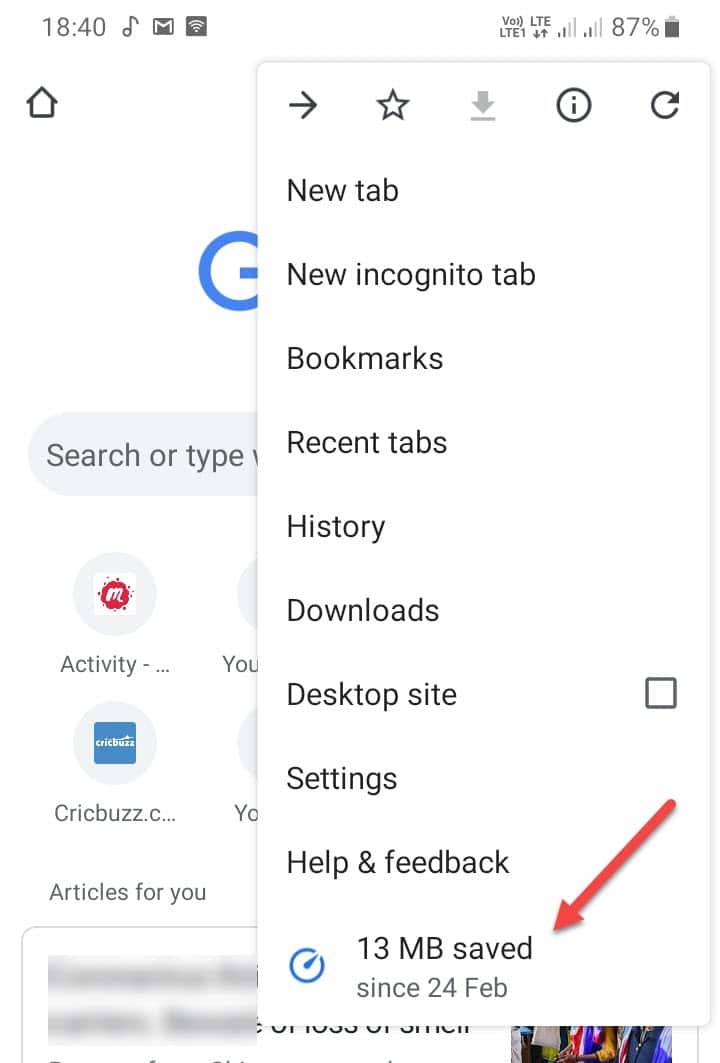The image is a screenshot taken from a smartphone. It is in portrait orientation with no defined borders but maintains the proportions of a phone screen. The top status bar displays various icons and information: the time "18:40" on the left, followed by a musical note icon, a Gmail envelope icon, and a Wi-Fi icon. To the right, it reads "VOLTE 1" next to an LTE icon with up and down arrows, a connection strength indicator showing two out of four bars, and a duplicate of the bars indicator. Further to the right, it shows "87%" alongside a battery icon with a black meter.

Below the status bar, on the left, is partially visible Google Home or search icon, specifically the blue "G" of the Google logo. The rest of the icon is obscured by a pop-up menu. This menu lists several options: "New Tab," "New Incognito Tab," "Bookmarks," and "Recent Tabs." At the bottom of the pop-up menu, there is a message in a horizontal configuration with a red arrow pointing to the left that states "13 MB saved since February 24," accompanied by a clock-like icon with a blue dial and border. This pop-up menu appears to provide quick access to common browser functions.